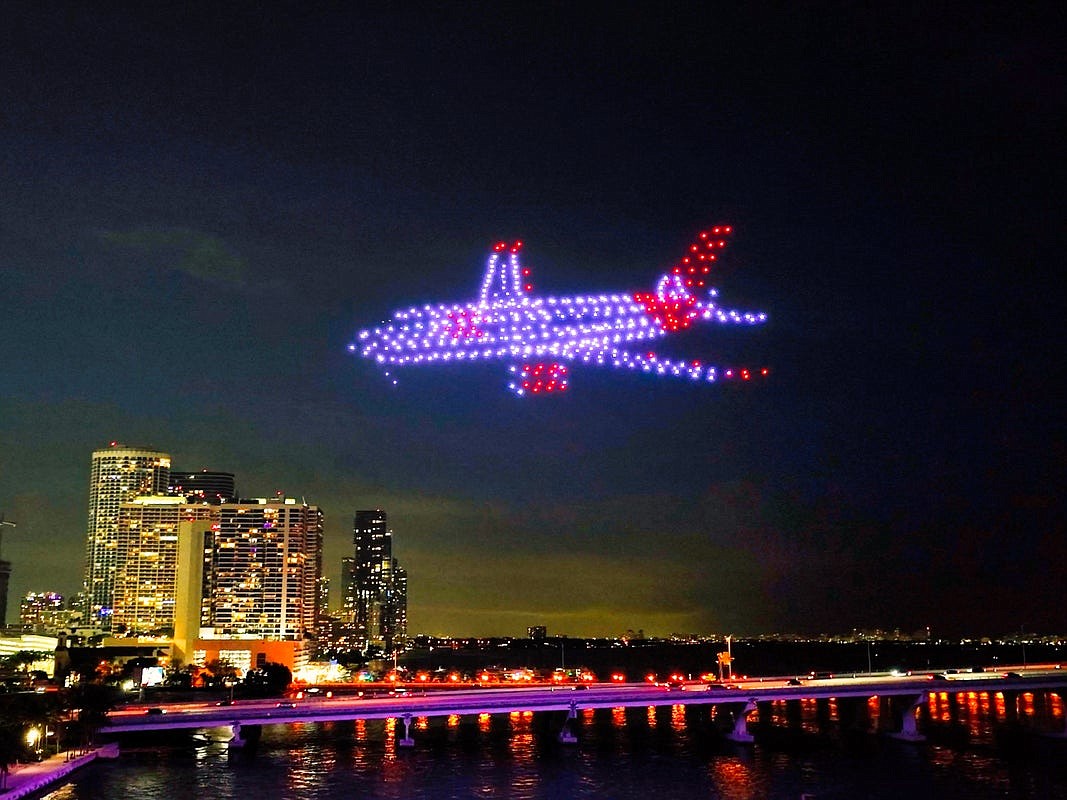This night-time photograph captures a vibrant cityscape illuminated against the darkness. Dominating the left side are towering, brightly lit skyscrapers that add a dynamic backdrop. In the foreground, a lit-up bridge spans a body of water, bustling with cars and tiny figures that hint at activity. The highlight of the image is dead center: a spectacular drone show. The drones, arranged to mimic the shape of an airplane, appear like a luminous aircraft made of Christmas lights. Primarily white with red accents on the tail, wing tips, and underside, the drones create a stunning, pixelated silhouette against the night sky. The scene is framed by city lights and the distant outline of more buildings, adding depth and context to this visually captivating urban tableau.